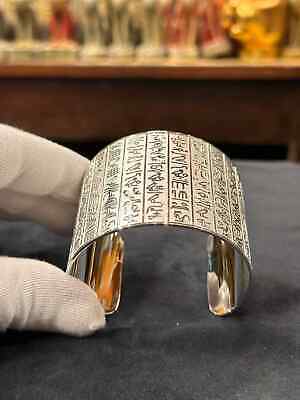An indoor image features a slightly blurred background showcasing a wooden shelf or cabinet adorned with colorful items in green, red, and gold. The gold item appears to be a small figurine. The focal point of the image is a white-gloved hand holding an ornate bracelet, possibly an ancient artifact. The bracelet, approximately 2 inches wide, is crafted from a silvery or white metal and is engraved with what appear to be hieroglyphics or abstract geometric patterns in gray. It has sections of gold bands with detailed engravings. The bracelet is displayed on a dark grey fabric surface.